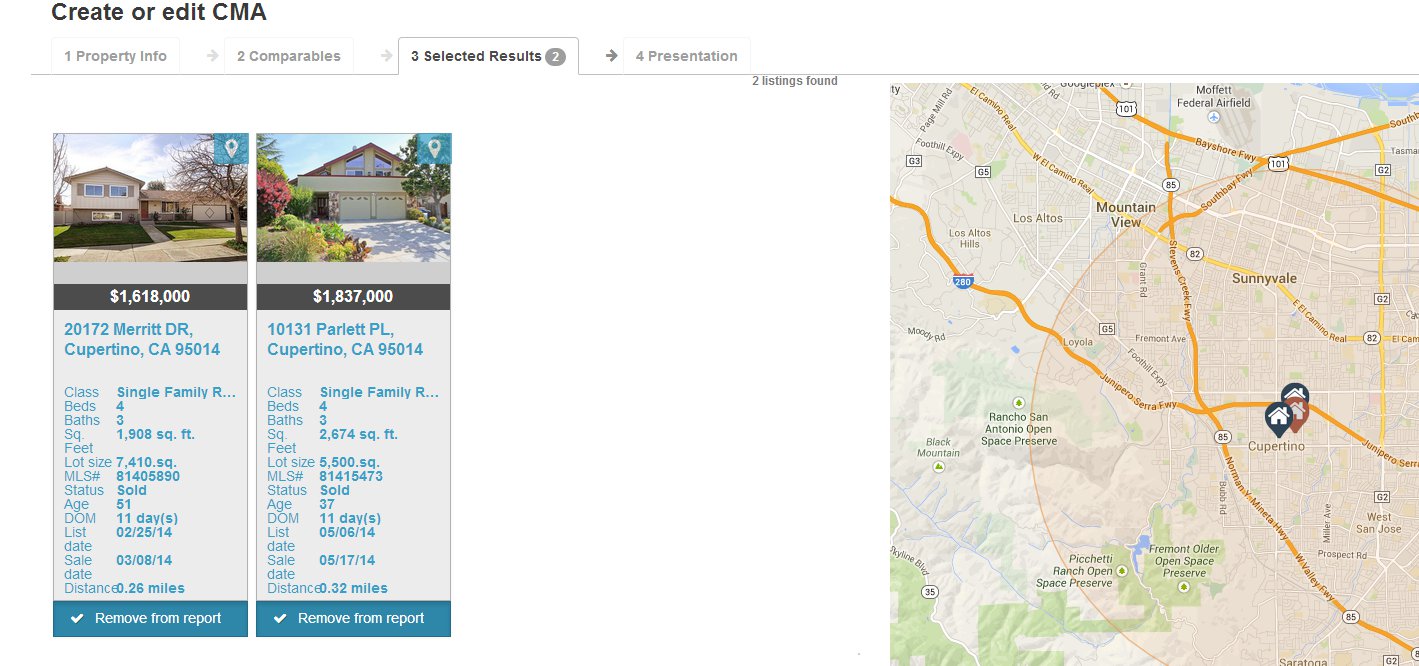The image depicts a real estate website interface designed for creating or editing Comparative Market Analysis (CMA) reports. At the top of the page, a prominent header reads "Create or Edit CMA," though the exact function is not immediately clear. Below the header, a navigation menu is segmented into four consecutive tabs labeled: "1. Property Info," "2. Comparables," "3. Selected Results," and "4. Presentation." A horizontal rule separates this menu from the main content area.

Beneath the rule, a text block announces the discovery of two property listings, each valued near $2 million. The first listing is priced at $1,618,000 and is located in Cupertino, California. This single-family home features four bedrooms, three bathrooms, and encompasses 1,908 square feet. The second listing, also in Cupertino, is priced at $1,837,000. It offers four bedrooms and three bathrooms as well, but its living space is significantly larger at 2,674 square feet.

On the right-hand side of the screen, an inset map displays markers pinpointing the locations of these two listings, providing a geographical context to their positions.